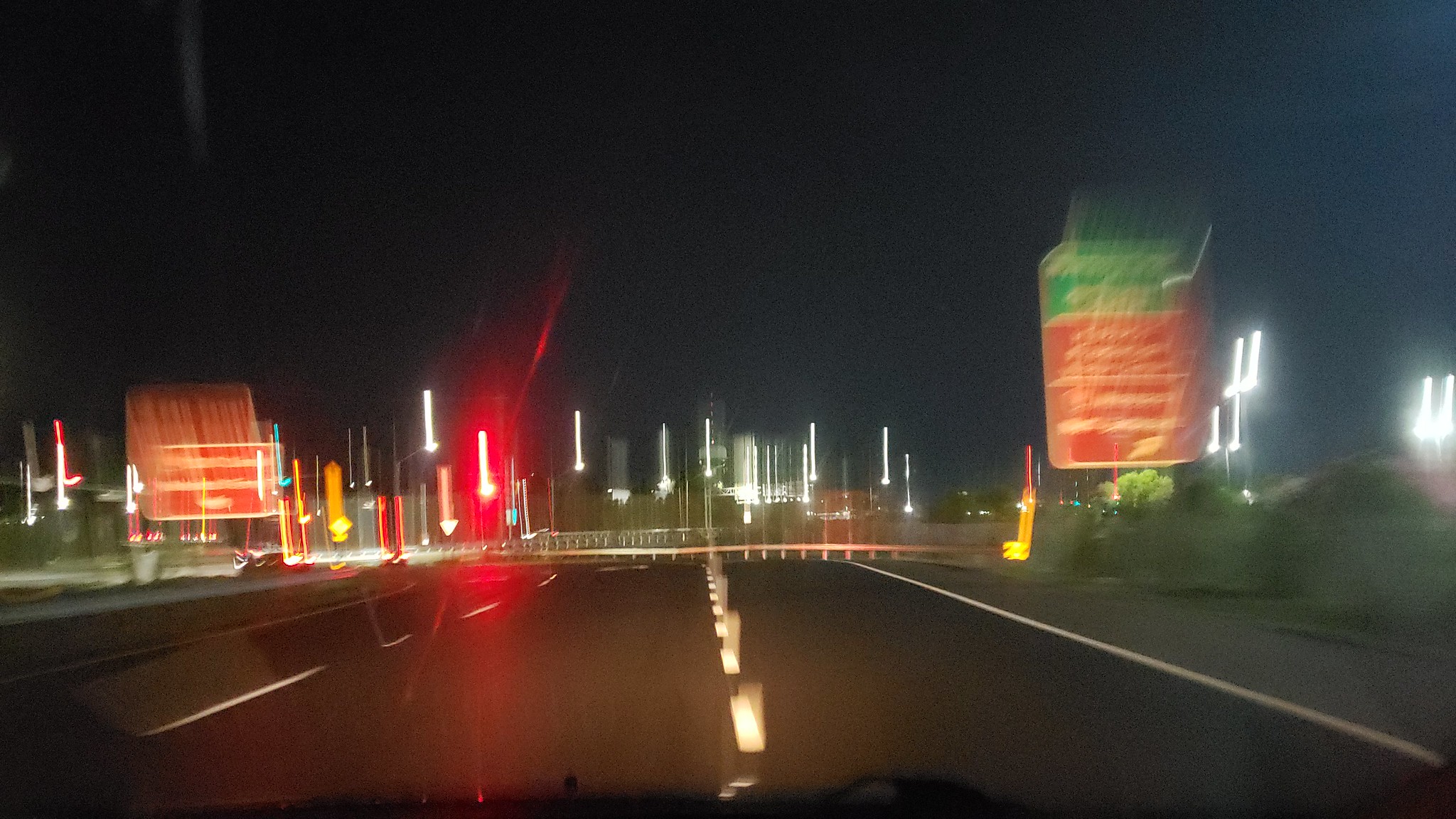A blurred photograph captures the view from inside a moving vehicle, situated in the middle of a freshly paved, black asphalt road. The slight disorientation from the blur suggests motion and imparts a dynamic quality to the image. On either side of the road, various signs are visible, likely providing directions or descriptions related to nearby buildings. The lights along the road appear distorted, resembling upside-down arrows due to the blurred effect. In the distant background, a singular building can be faintly discerned, standing as the apparent destination towards which the road leads. The overall scene focuses on the journey down this clear, newly constructed road, with the blurred elements adding a sense of speed and movement.